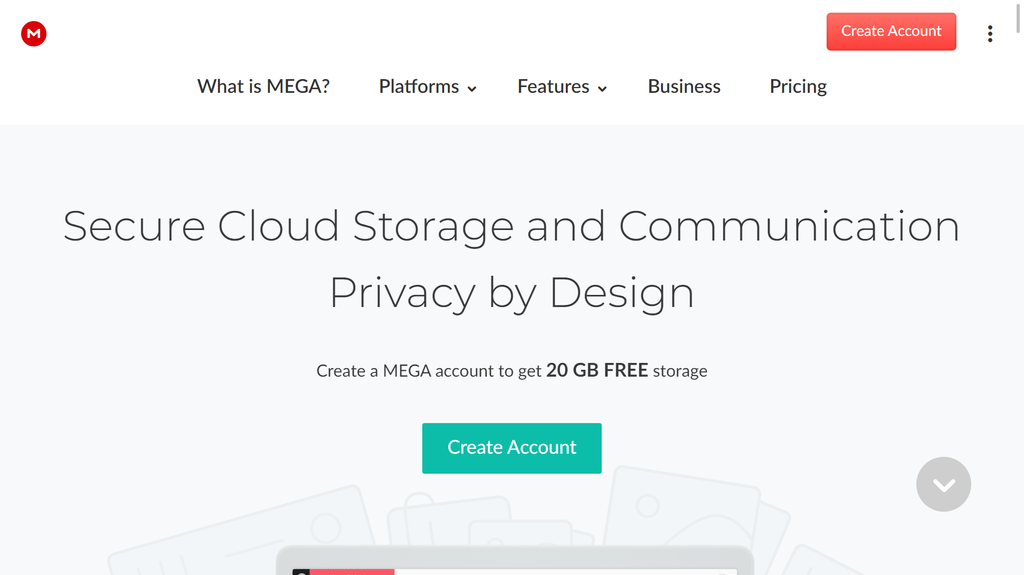In the image, the upper left corner features a white "M" within a red circle. On the right side, there is a red button with white text that reads "Create Account." Adjacent to it, three vertical black dots serve as a menu or settings icon. Beneath this section, bold text asks, "What is MEGA?" followed by "Platforms," "Features," and "Business Pricing," each accompanied by a dropdown menu.

The background transitions to a lighter gray hue below these elements. Dominating this area is the largest text in the image: "Secure cloud storage and communication privacy by design." Below, a call-to-action states, "Create a MEGA account to get 20 gigabytes of free storage," highlighted by a teal button with white text that reads "Create Account." To its right, there is a gray button with a white drop-down arrow, suggesting additional options.

Near the bottom, the image includes a horizontal gray line with sections in red (left), white (middle), and another indeterminate color, likely due to the lower part being cut off. The primary colors evident in the design are red, white, black, gray, and teal green. The context suggests it could be a webpage or a tablet interface in horizontal orientation, but no definitive URL or specific format details are provided.